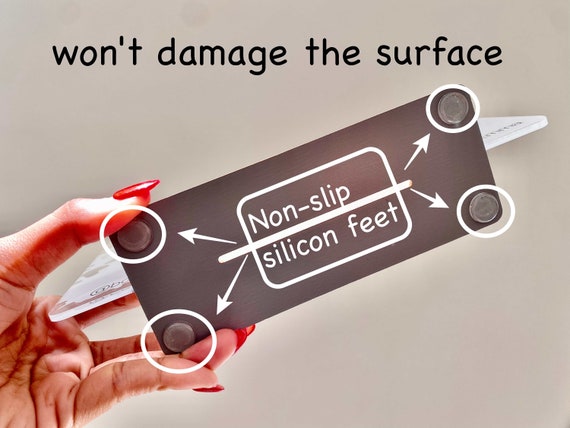The image depicts an advertisement featuring a woman’s hand with bright red, well-manicured fingernails, emerging from the lower left corner. She is holding up a black, rectangular object with slightly wrinkled palms. The background is a plain white color, accentuating the central focus on the object and text. At the top of the image, “Won’t Damage the Surface” is prominently displayed in black font. Below, white text labels four transparent, coin-like pegs on each corner of the object's base as “Non-Slip Silicone Feet,” underscoring the product's non-damaging and stable design. Behind the object, subtly visible, is a plate. The overall composition suggests that the object is likely a tray with a clear glass or display case on top.